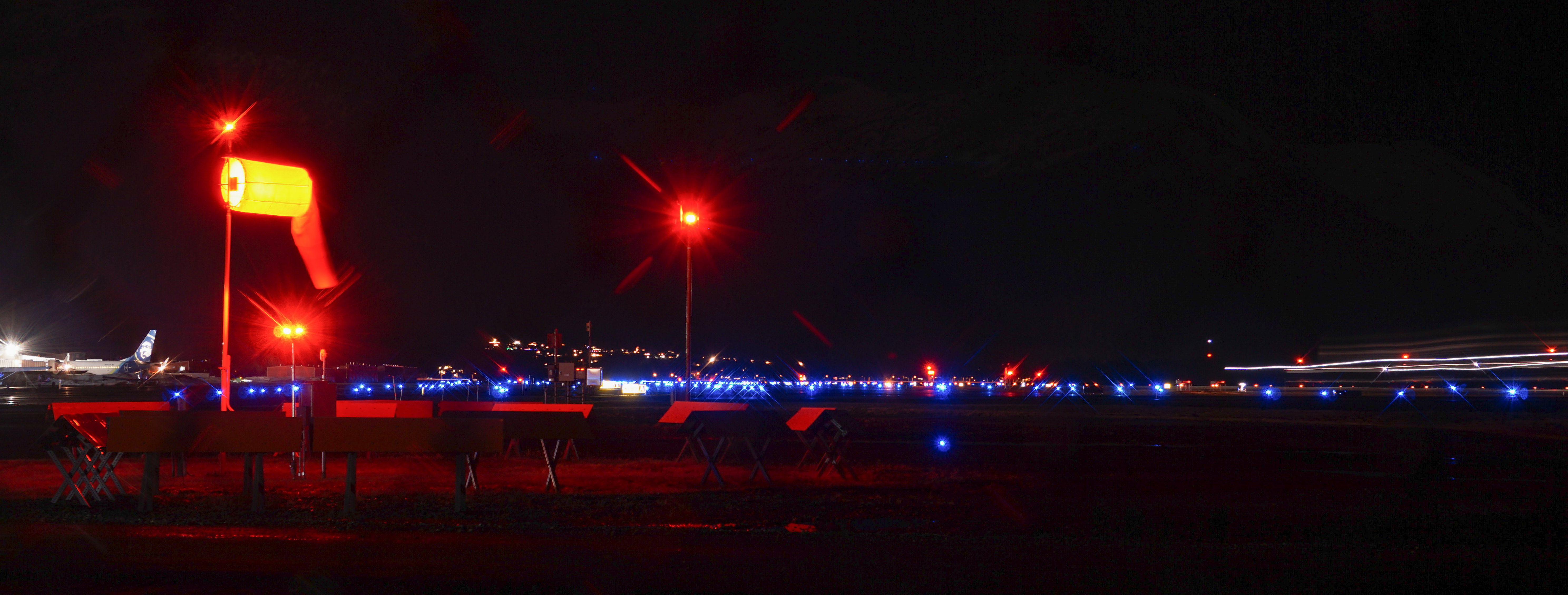This image depicts a nighttime scene at an airport runway. Dominating the left side is a large, parked white airplane with a blue tail. Adjacent to it, several air cranes are stationed. The runway itself is festooned with numerous blue and red lights, occasionally interspersed with goldish hues, clearly marking the path for arriving and departing aircraft. In the foreground stands a cylindrical flag, partially caught by the wind and illuminated by bright red lights above and below it. Nearby are other structures likely supporting signage or light reflectors. 

Toward the center, an intensely glowing red light stands out, resembling a lollipop in its vibrancy, and is one of three such striking red lights that color the surrounding area with their glow. The middle section of the image showcases a horizon line populated with mostly blue lights, hinting at the organized layout of the runway. Additionally, there is a circular area featuring solar panel-like structures, lit by red lights which give this section an intriguing appearance. In the distant background, the faint lights of a cityscape and a few electrical wires are visible under the dark, moonless sky, contributing to the overall portrayal of a quiet, yet bustling night at the airport.